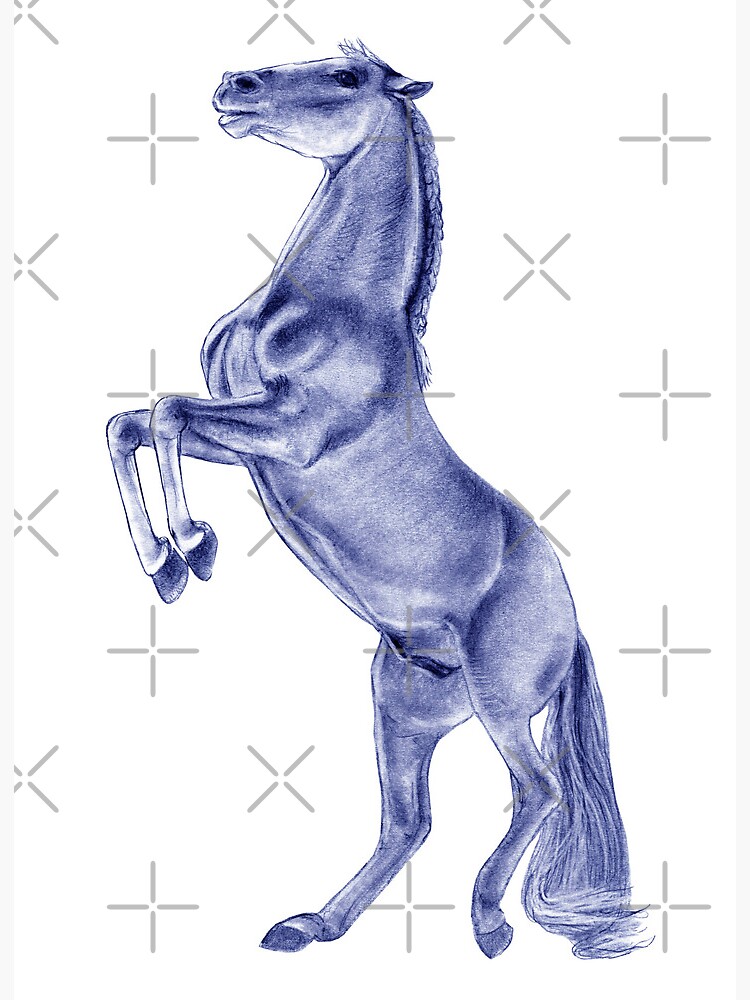The image showcases a detailed drawing of a horse, rendered in colored pencil with a sophisticated blend of white and various shades of blue, almost transitioning into purple in some shaded areas. The horse is depicted rearing up on its hind legs, creating a vertical composition with its front legs folded upwards. The mane, intricately braided around its head, and the long tail, which touches the ground, add to the horse's regal posture. The horse has a distinctive black eye that stands out against its lighter body tones.

In the background, there is a pattern of gray crosses against a white backdrop. The crosses consist of simple intersecting lines, arranged in a grid where their orientation alternates between columns—some are turned 45 degrees to form diagonal Xs, while others stand straight. This intricate background provides a contrasting yet complementary setting for the illustrated horse, enhancing the overall visual appeal of the artwork.